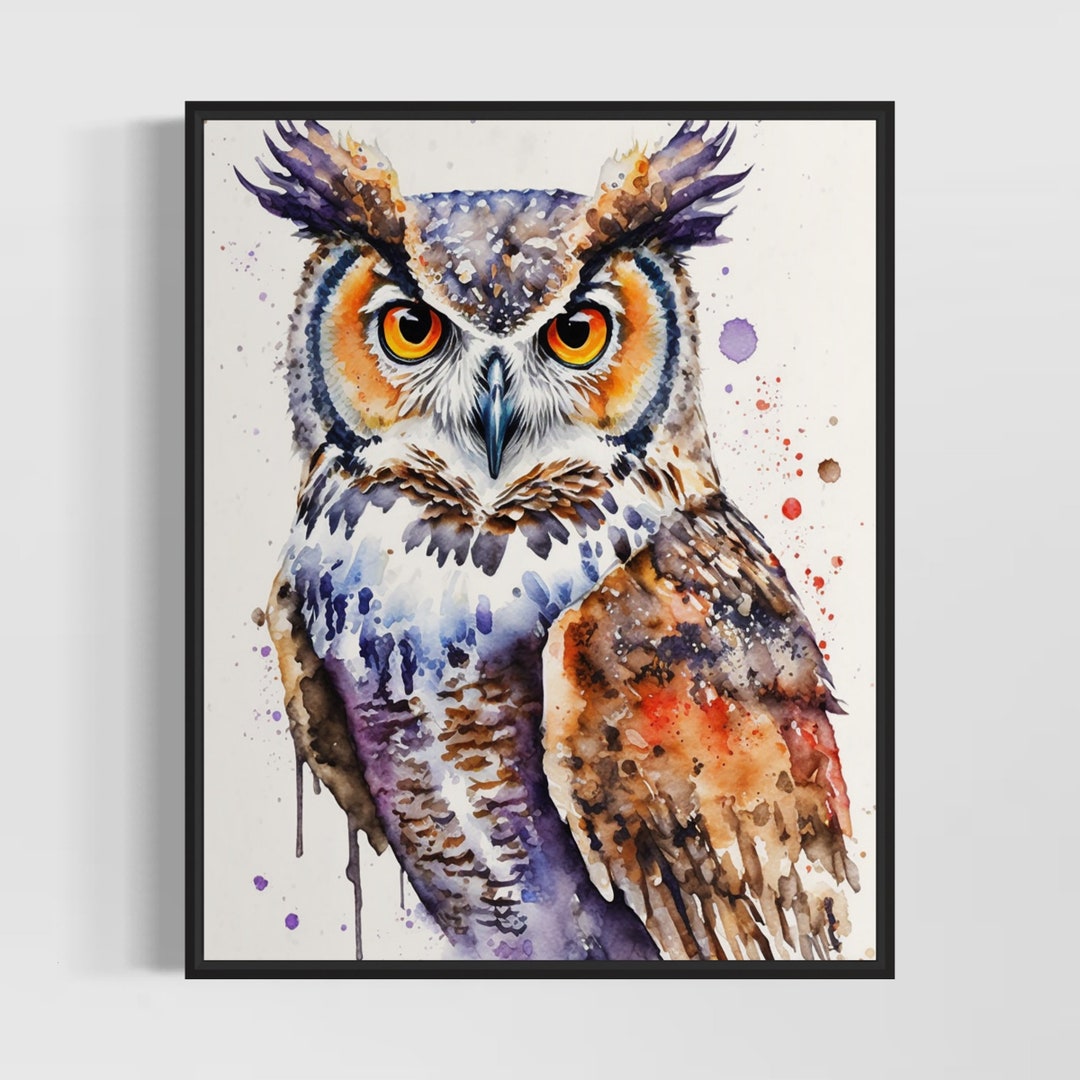The photograph showcases a framed print prominently displayed in the center against a light gray wall. This print features a stunning watercolor or gouache and pen and ink illustration of an owl, rendered with exquisitely soft washes to highlight the intricate details of its feathers. The owl, occupying most of the image, captivates with its vivid, bright orange eyes that gaze directly at the viewer. The artist employs a rich palette, combining shades of orange-red, purple, purplish-blue, gray, brown, and white to breathe life into the owl's plumage. The bird's right wing extends to fill the bottom right portion of the frame, adding depth to the composition. The background is subtle yet dynamic, adorned with delicate speckles and tiny bubble-like splatters that enhance the visual interest of the artwork. The framed print casts a gentle shadow to the left, further defining its presence on the wall.